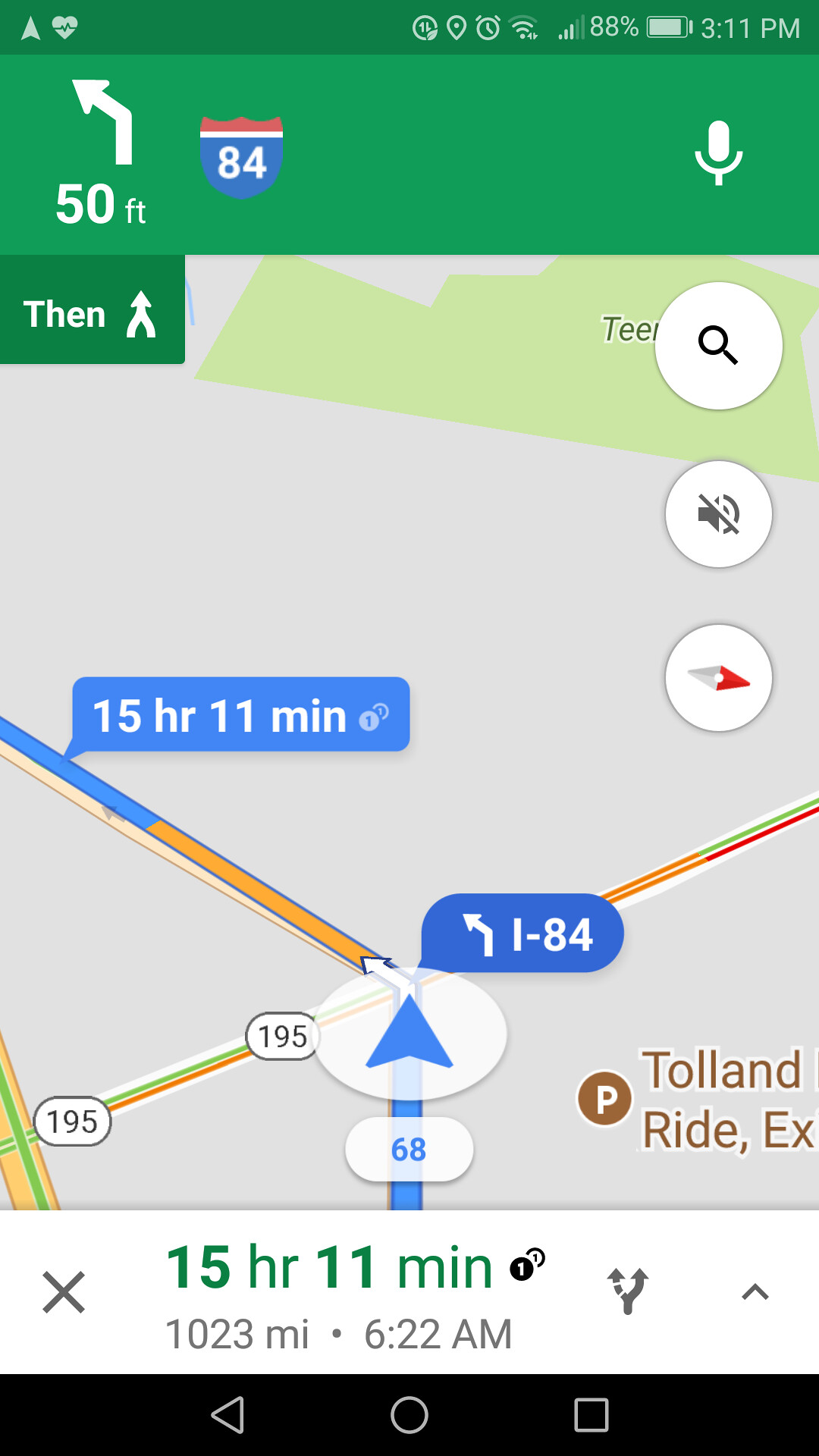The image is a screenshot from a phone's navigation app taken at 3:11 PM with 88% battery remaining, as indicated by the icons at the top of the screen. The map centers around a route to a destination that is 1,023 miles away, estimated to take 15 hours and 11 minutes to reach. A key landmark displayed on the map is Toland Ride EX. The navigation shows the user’s current position marked by a blue arrow encircled, and their route is highlighted in blue. There are clear indicators of turns, such as a left turn onto I-84, which is displayed in a white-on-blue bubble, and the information is emphasized with additional directional cues. The freeway, also displayed on the map, aligns with routes like Highway 195. The detailed map interface highlights real-time navigation with comprehensive travel instructions.